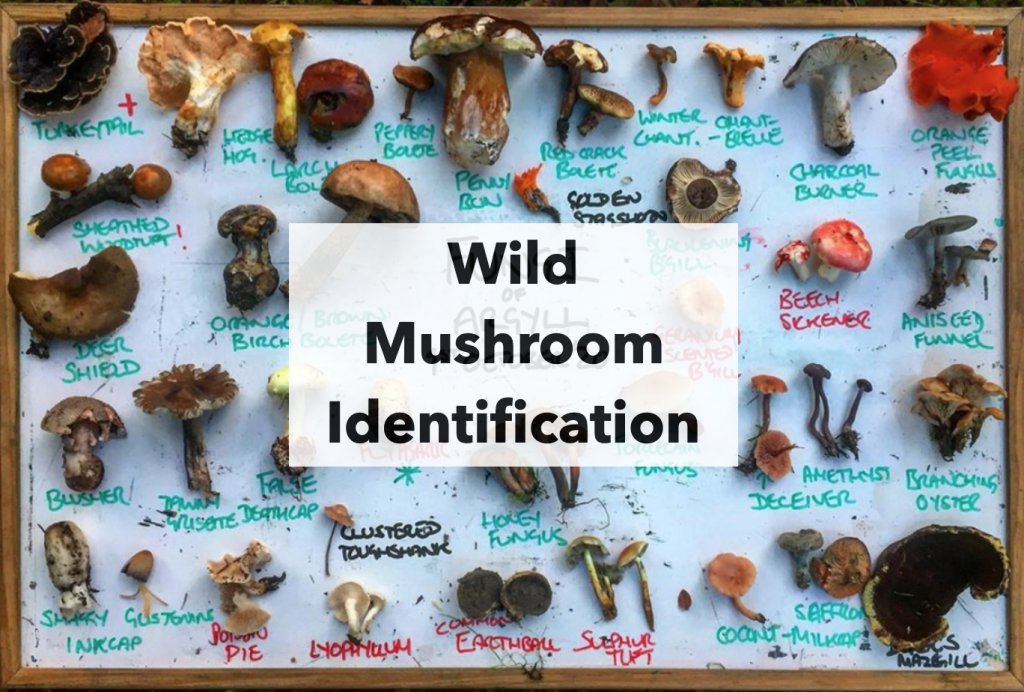Detailed Description: 

The image showcases a wooden-framed display with a light blue background, possibly paper or a whiteboard. The wooden frame is surrounded by thin wood trim. Inside the frame, various types of mushrooms are arranged in neat rows, spanning from left to right. Each mushroom is meticulously labeled underneath, with names written in either green, purple, red, or black ink. 

In the center of the display, a white rectangle is superimposed, bearing the title "Wild Mushroom Identification" in black text, with each word on a separate line. The mushrooms themselves vary in color, including orange, brown, black, pink, and red. Notable mushrooms include one at the top labeled "turkey tail," which resembles an actual turkey tail, and another to the right labeled "hedge hog."

This organized chart effectively provides a detailed identification guide to different wild mushrooms, with clear and colorful labeling that assists in distinguishing each variety.